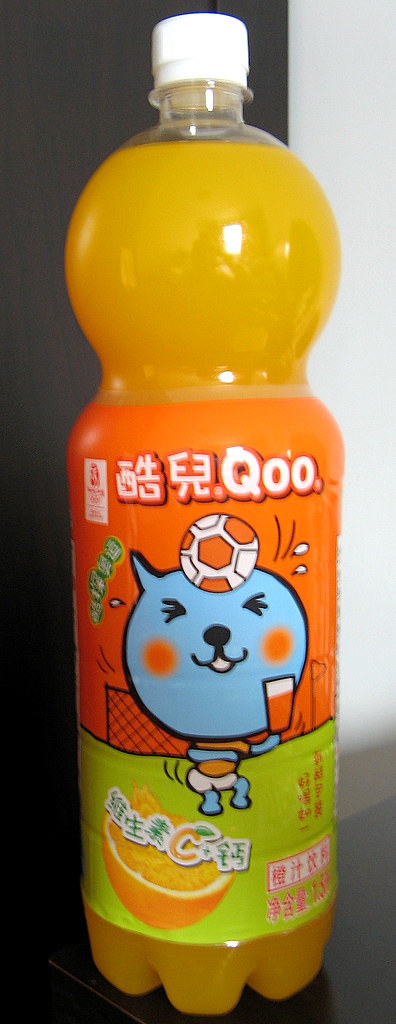The image depicts a portrait-style photograph of an orange beverage bottle, prominently placed against a black wooden background. The bottle itself is clear plastic with a white screw cap, containing an orange liquid that could be juice or soda. The bottle features a unique design: while the bottom has a typical shape with a textured, bumpy surface, the upper part is large and round, tapering into a neck beneath the cap. The label is vibrant and detailed, dominated by a large blue-headed cat with a disproportionately small body, humorously depicted with a soccer ball bouncing off its head. The cat is in front of a soccer goalpost, holding an orange cup, presumably filled with the same orange beverage. Surrounding the cat are elements like a whole orange and a slice of orange, with the distinctive letter 'C' and green Asian symbols inscribed within. The label's text is entirely in foreign, likely Asian, characters, underscoring the beverage's international origin.